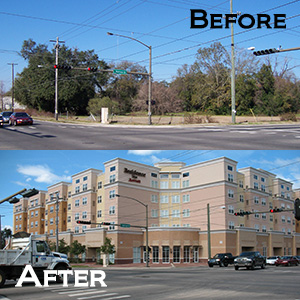The photograph is a composite of two rectangular images, one stacked above the other, each labeled "before" and "after" respectively. Both images were taken during the day, with clear blue skies and minimal clouds. The "before" image, marked by black text in the upper right corner, captures a vacant city lot at the intersection of two streets, featuring light poles, telephone poles, and several cars on the road. The lot is predominantly occupied by trees and bushes, indicating an underdeveloped area. 

In contrast, the "after" image, labeled in white text at the bottom left, showcases a prominent transformation. The once vacant lot now hosts a large building, which appears to be a four or five-story hotel, likely a Marriott, identifiable by its cream and salmon-colored facade and intricate entrance boasting multiple doors. The building's windows are decorated with white trimming. The traffic seems heavier in this image compared to the "before" image, with more cars visible on the streets. The significant redevelopment of the intersection is highlighted by the stark difference between the two photos.